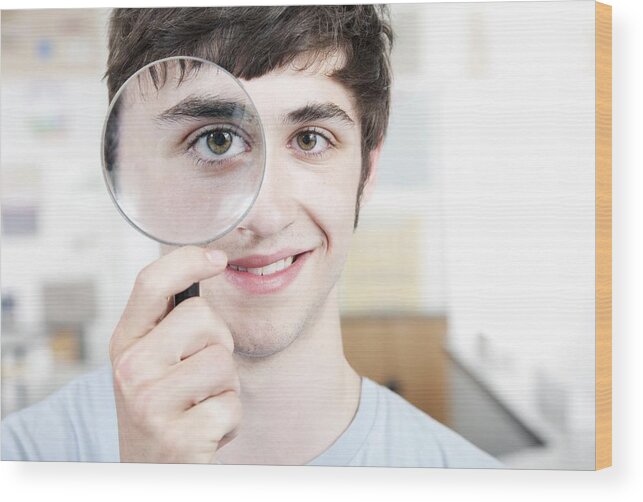The photograph showcases a young white man grinning as he holds a black magnifying glass up to his right eye with his right hand, causing his right eye to appear vividly magnified. He has short dark brown hair combed to the side, thick brown eyebrows, brown eyes, and a hint of beard growth along with longish sideburns. He is wearing a light gray t-shirt. The background suggests a classroom or a hallway adorned with blurry, colorful items against white walls. The image is printed on a textured canvas, lending it a textbook or magazine quality with wooden edges. The setting remains indistinct but hints at an educational setting due to the visible items on the walls.